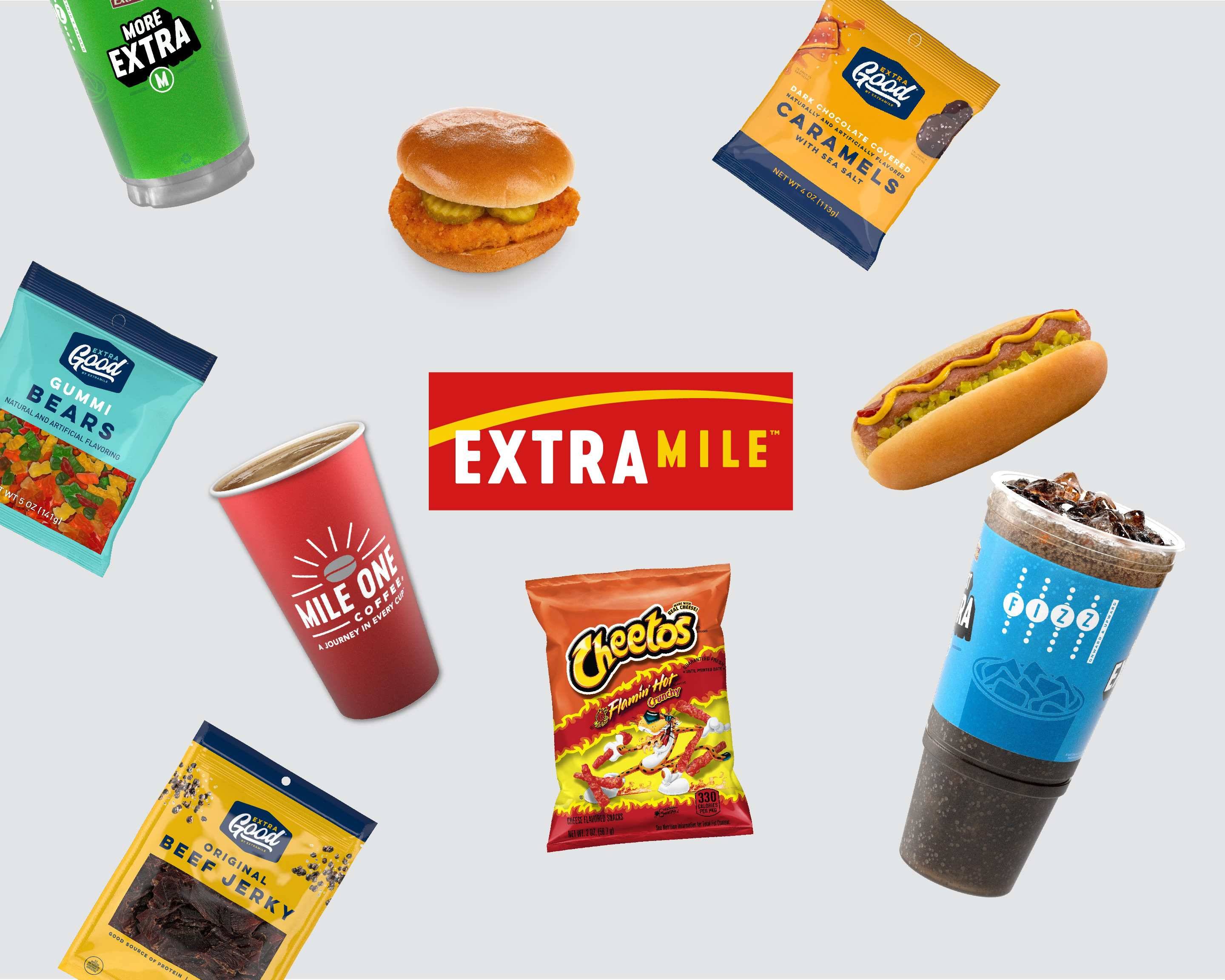This image appears to be an advertisement, likely for a convenience store or a specific brand called "Extra" which is prominently displayed on a central red banner with a yellow swoosh, featuring the words "Extra Mile." The backdrop is light gray, creating a neutral setting for the items showcased. Arrayed around the banner are various food items, predominantly of the "Extra" brand, presented in a clockwise arrangement from the top left. 

Firstly, there is a green item partially cut off in the top right corner labeled "More Extra." Following this, there's a chicken sandwich with two dill pickle slices peeking out. Next, there is a bag of sea salt caramels. Continuing clockwise, we see a hot dog topped with a colorful trio of ketchup, mustard, and relish. Moving on, there's a large soft drink filled with ice cubes, likely Coke or Pepsi. At the six o'clock position, a bag of Flamin' Hot Cheetos can be seen. Below this, near the bottom left is a bag of Original Beef Jerky. Upwards near nine o'clock is a red "Mile One" coffee cup with a white rim. Finally, there's a bag of gummy bears.

The image is detailed and vivid, evoking the look and feel of a store display or a low-budget advertisement—possibly designed for social media or print mediums such as the back of a magazine. The cohesive brand theme emphasizes convenience and variety, encapsulated by the "Extra Mile" banner at the core.